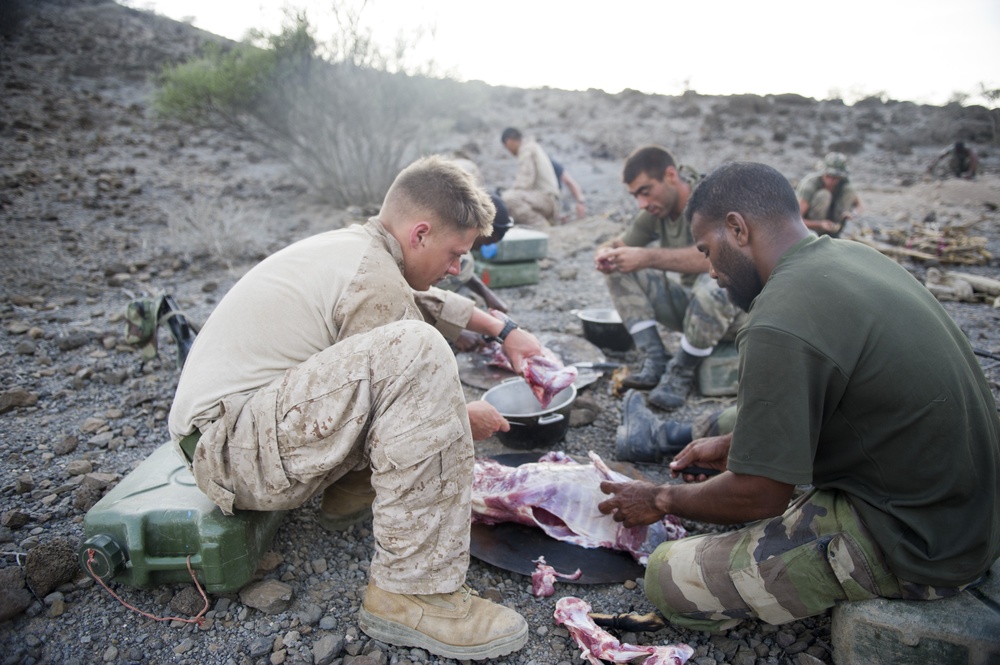In this detailed horizontal photograph, a group of soldiers is depicted in a dry, barren, rocky landscape with minimal vegetation, save for some weedy plants and a sparse, slightly green tree in the background. The central focus is on three soldiers seated in a semicircle around a large chunk of raw meat placed on a black tray. One soldier on the left, dressed in tan army fatigues and tan boots, is leaning over a pot, seemingly preparing the meat for cooking. Another soldier on the right, dressed in darker green and olive camo fatigues, is cutting strips of the meat with a knife. They are sitting on rocks and various makeshift seats, like canteens and fuel tanks.

In the background, more blurred soldiers can be seen, also attired in a mix of tan and green military uniforms, contributing to the food preparation. The setting is indicative of an arid, hilly area, with a hill on the top left and some sparse leaves and shrubs. The photograph captures a moment of pause in the soldiers' day, possibly a break for lunch, emphasizing the raw meat being prepared and the soldiers' collaborative effort in a challenging environment.